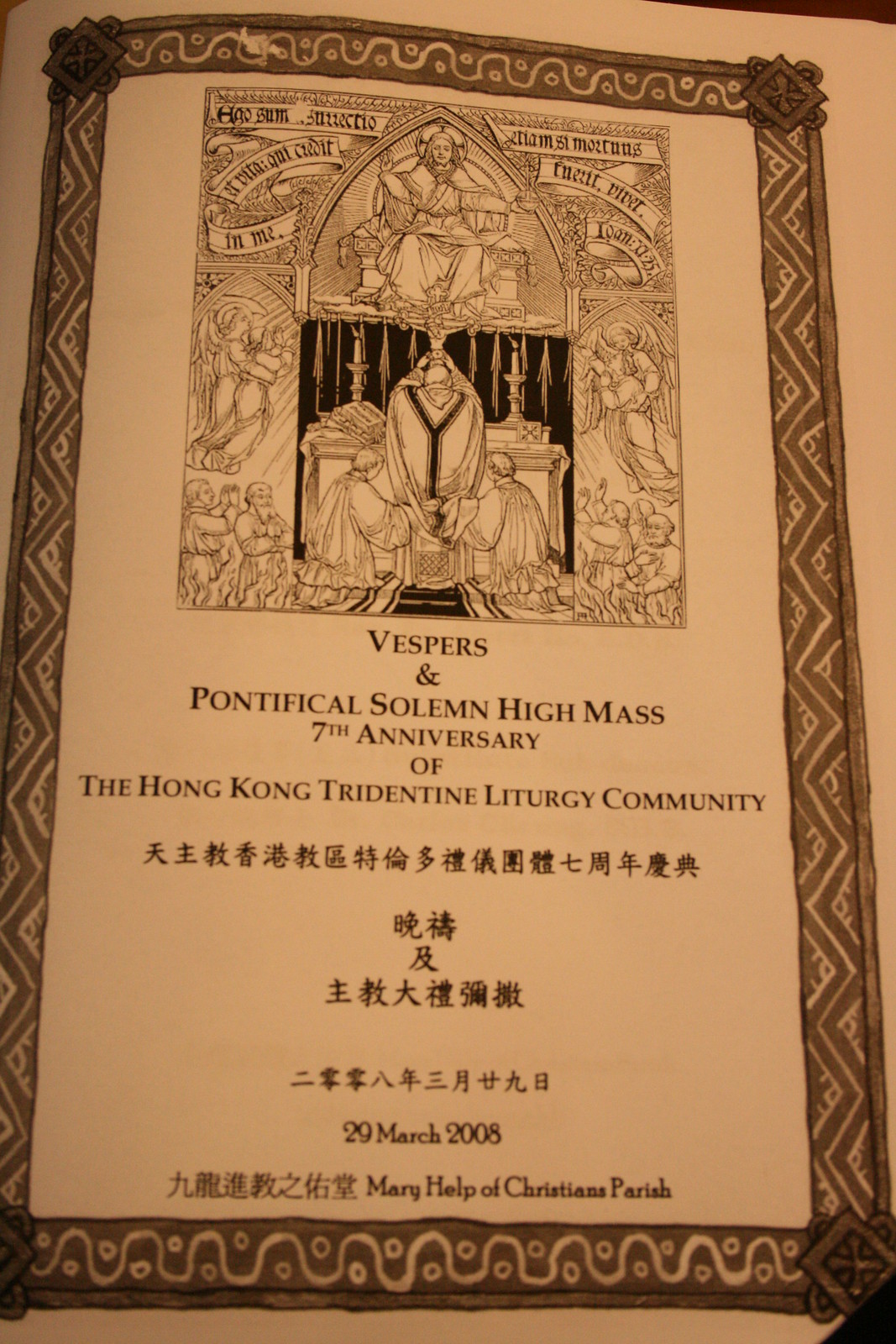The image depicts a vertically oriented, rectangular page, likely from a book or a specialized religious program. The page has a light brown hue and is encased within an intricate, thick, zigzag-patterned border. Centered at the top of the page is a detailed, square-shaped drawing depicting a woman seated on a throne with a man sitting below her, attended by two servants. The text beneath this illustration reads, "Vespers and Pontifical Solemn High Mass, 7th Anniversary of the Hong Kong Tridentine Liturgy Community," presented in brown, all-caps text. Below this central inscription is a row of symbols, followed by three additional lines of similar symbols, and another row of symbols at the very bottom of the page. The date "29 March 2008" is featured prominently above the final set of symbols, which are accompanied by the inscription "Mary Help of Christians Parish," suggesting a Catholic service setting. The overall aesthetic and design evoke a medieval or mid-century church service program, possibly written in Latin, with additional notation in Chinese characters. The primary colors in the image include brown, black, white, and gray.